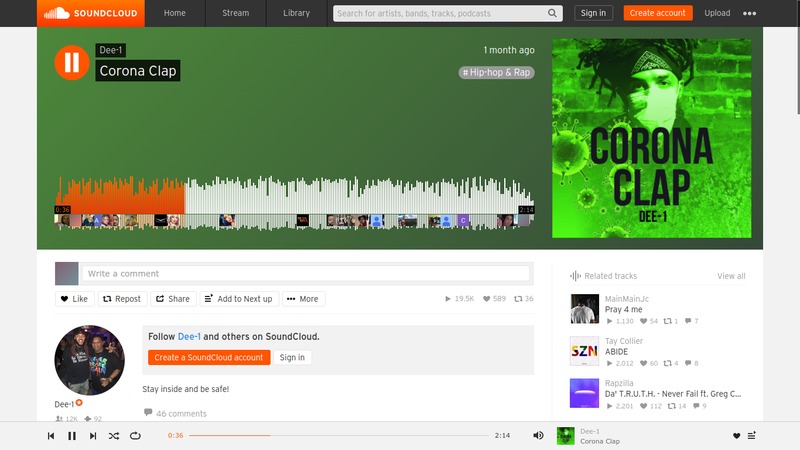This image is a screenshot of a SoundCloud page showcasing the artist D1's track titled "Corona Clap." Dominating the screen is the large banner displaying the artist's name, D1, and the song title, "Corona Clap," signifying that the song was posted a month ago under the genre of Hip Hop and Rap.

On the right side of the screen, there is intriguing cover art featuring a person standing against a brick wall. The person is wearing a mask and has a bandana tied around their forehead, with dreadlocks peeking out from the top. The cover art has a green tint overlay with floating virus-like images, creating a vivid thematic representation of the song's title. Below the image, the text "Corona Clap D1" is displayed.

At the bottom of the screen is a functional section where users can interact with the track by writing a comment, liking, reposting, sharing, or adding it to their "next up" queue. There is also a "more" menu for additional options. Users can see the icon of the artist or the poster and have the option to follow D1 and other artists on SoundCloud. There's a visible comment from a listener stating, "stay inside and be safe."

On the bottom right of the image, there is a section titled "Related tracks" featuring a list of three other artists and their song titles in small font. The very bottom of the screenshot includes playback controls such as the pause button, previous track, next track, shuffle, loop, the song's progress bar, volume control, and once again displays the artist’s name and song title.